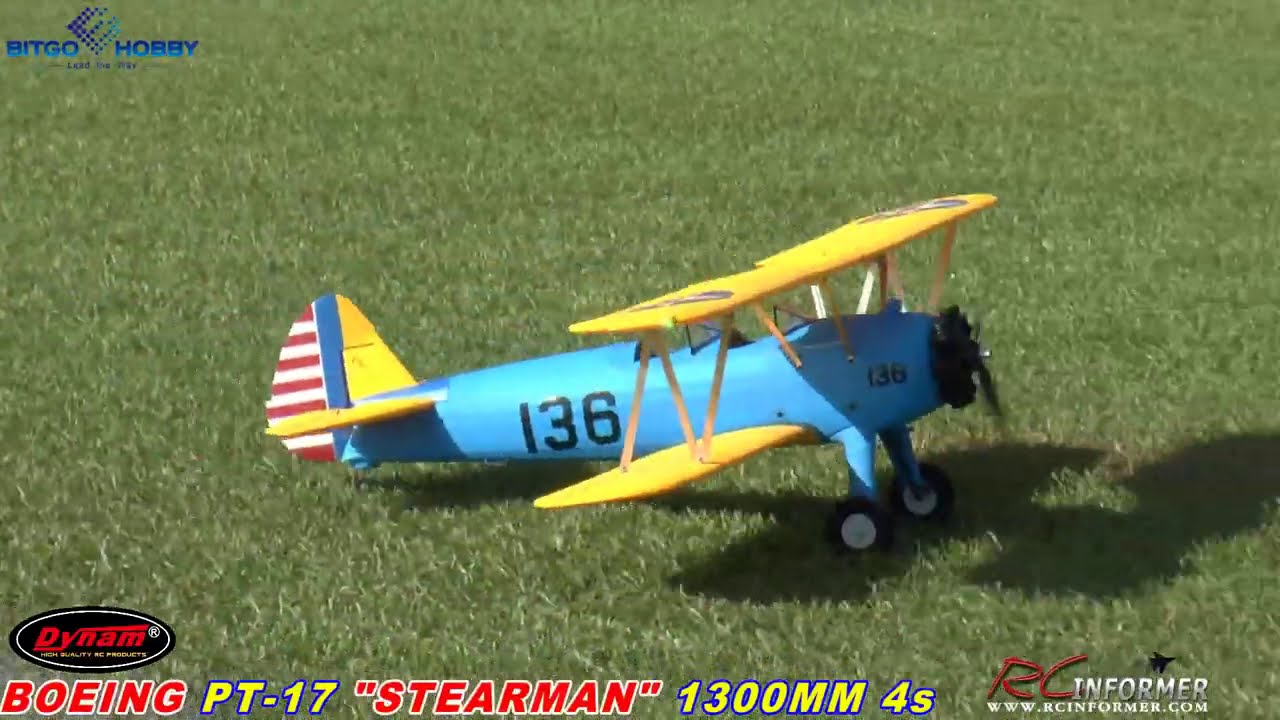This high-definition image showcases a detailed model airplane, specifically a vintage Boeing PT-17 Stearman. The plane's body is painted a light sky blue, while its wings and tailfins are bright yellow. It embodies the classic biplane design, with one set of wings positioned above the other. The tail features a mix of colors, including a vertical fin with a blue stripe and alternating red and white horizontal stripes. At the nose, there's a black propeller that appears to be in motion. The plane sits on grass, adding a lifelike touch to the scene.

The plane prominently displays the number 136 in black near the front propeller and along its fuselage. The landing gear has black tires with white hubs. Various labels and logos are visible: the BitGo Hobby logo is in the upper left corner, and along the bottom, text details the model's specifications. In a black oval with red letters, it says "DYNAM," followed by "BOEING" in red, "PT-17" in yellow with a blue outline, "STEARMAN" in red within quotes, and "1300MM 4S" in yellow with a blue outline. Additionally, "RCInformer" appears in red and white next to the website address "www.rcinformer.com."

This comprehensive composition not only highlights the intricate design and vibrant colors of the model airplane but also provides insight into its branding and scale, making it clear that this is a cherished piece, likely used by hobbyists and aviation enthusiasts.